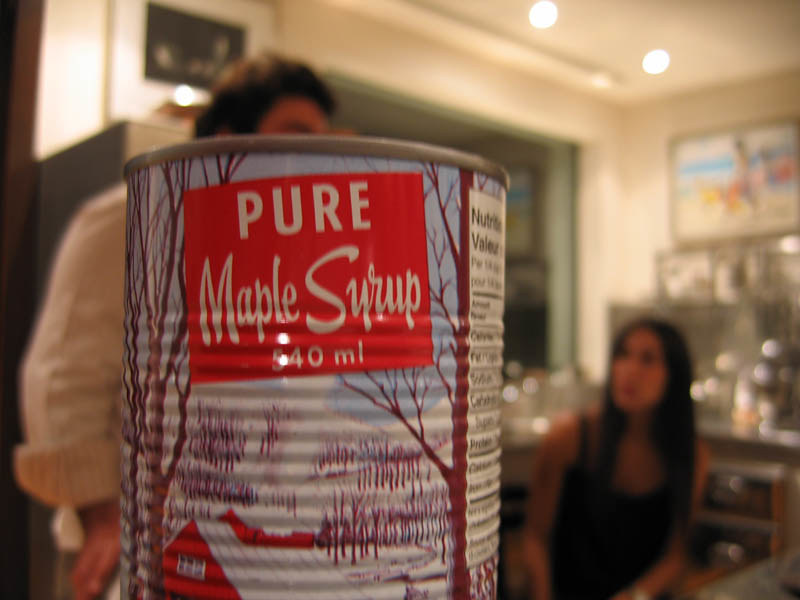The close-up photograph prominently features a can of pure maple syrup, labeled with a volume of 540 milliliters. The can's design includes an illustration of a snowy scene. To the right side of the can, a portion of the nutrition values is visible, though the text is unreadable as the label is turned away. The photo suggests that the can is being held up by the photographer. 

In the background, two individuals are visible but blurred and out of focus, emphasizing the can as the main subject. A man is standing directly behind the can, while a woman is seated, looking up at him. The background, likely a kitchen area, includes what appears to be a metal sink behind the woman, adding context to the setting.